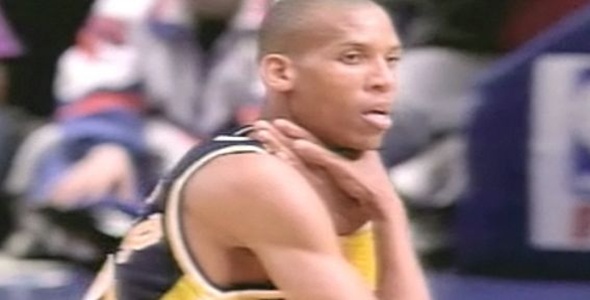The image appears to be a screen capture of an old broadcast, showing basketball player Reggie Miller seemingly mimicking a choking gesture. Both of Miller's hands are positioned around his neck, with his left hand underneath the right. His mouth is open, revealing both rows of his teeth, and he gazes into the distance. Miller's posture appears slightly bent, suggesting a squatting or seated position. He is notable for his very short dark hair and is wearing a blue, white, and yellow sleeveless jersey. The scene behind him is quite blurry, only hinting at the presence of a crowd with indistinct colors of blue, white, and red. The quality of the image is notably low, probably a result of being recorded onto tape and then captured as a screenshot. The frame cuts off the top of Miller's head and ends not far below his armpits.